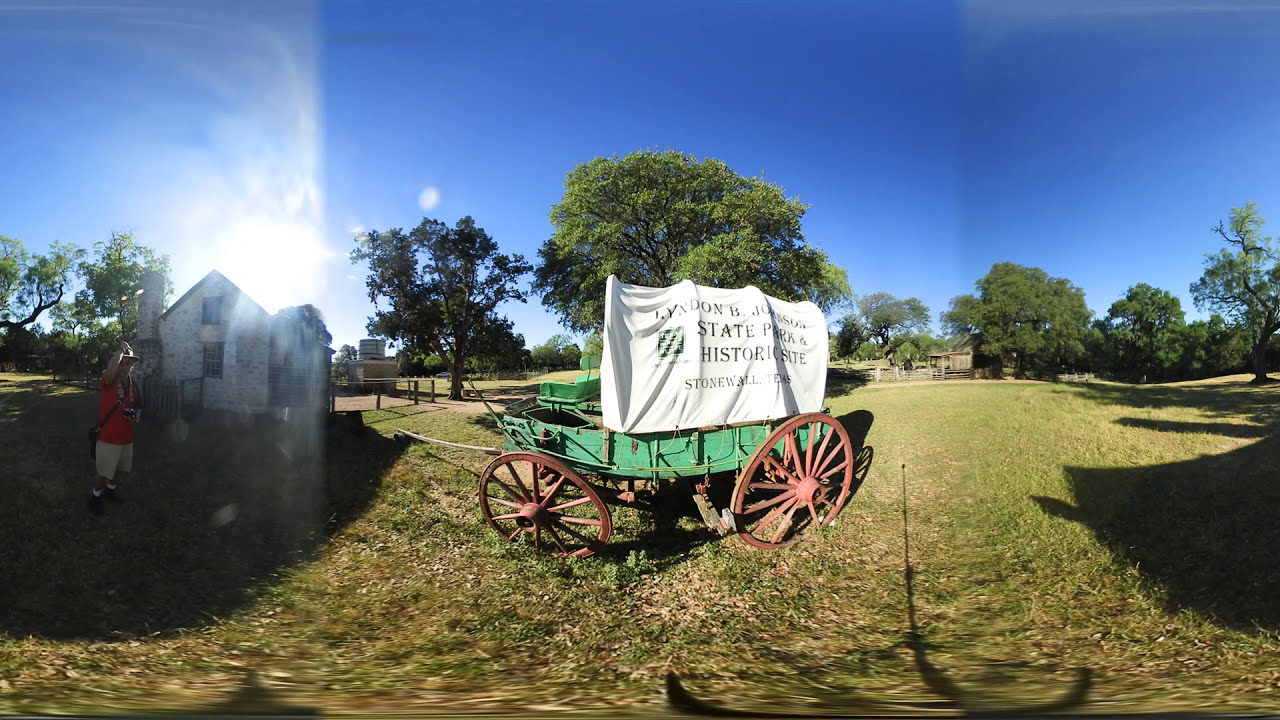In this image, a green covered wagon sits prominently in an open grassy field, centered within the frame. The wagon, with red wheels and a canvas cover that reads "Lyndon B. Johnson State Park and Historical Site, Stonewall, Texas," is framed against a backdrop of clear blue skies and sparse clouds. The photo includes elements indicative of a sunny, midday setting. To the left of the wagon stands an older man wearing a red shirt, white shorts, and a cap, positioned near a small two-story stone or brick house with a chimney. The location appears to be an outdoor state park with historical significance, characterized by scattered trees and distant fences contributing to the pastoral ambiance. The image seems to be a panoramic shot, leading to slight distortions and large shadows due to the sun's low angle. No text or signage is visible other than on the wagon's canvas. The scene is serene, with colors including various shades of blue, green, red, and orange woven throughout.